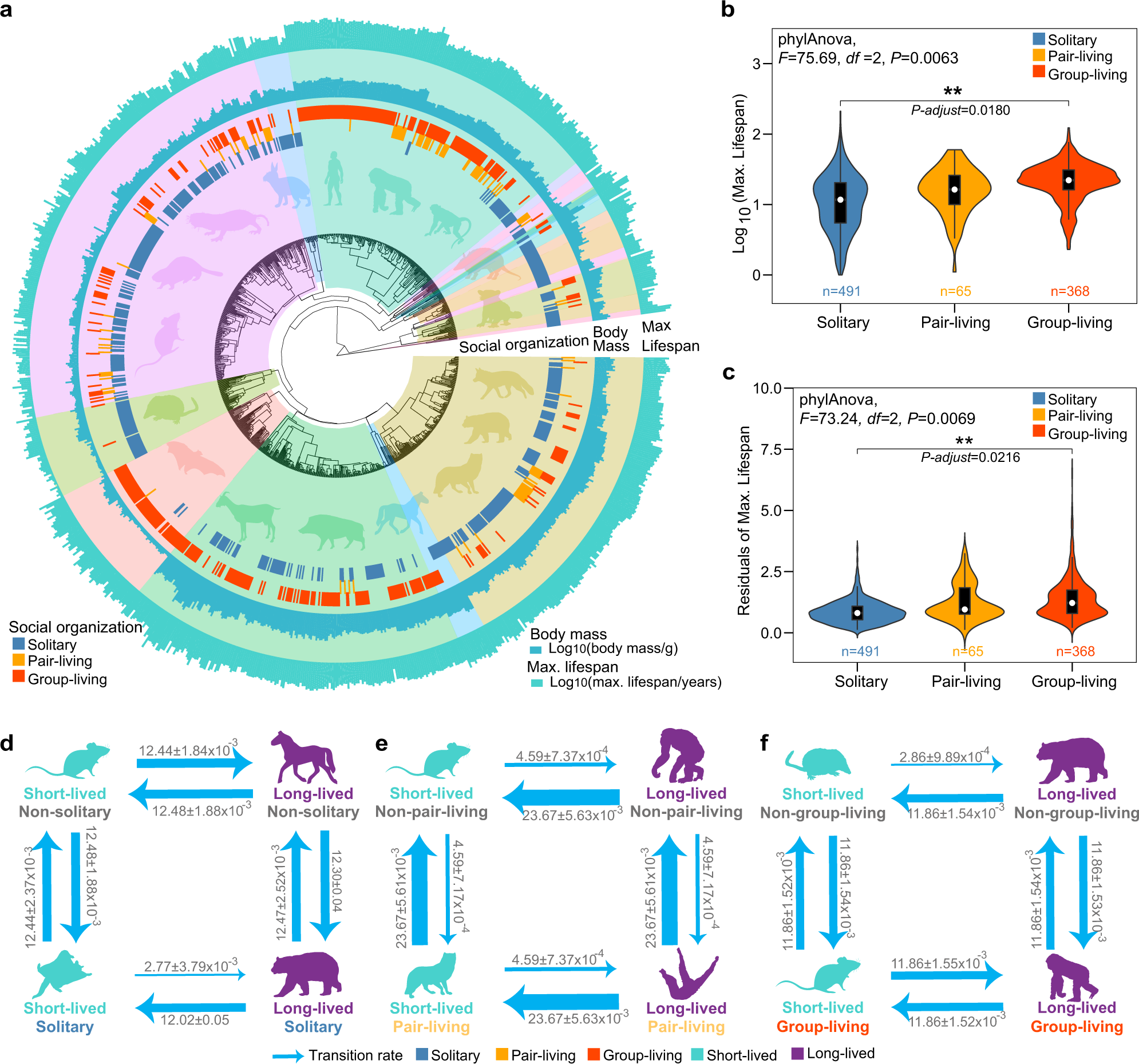This detailed and informational graphic is presented on a white background and is divided into four main sections, labeled from A to F in black text. 

In section A, located in the top-left corner, there's a circular bar graph with concentric circles in black, blue, orange, and green. In the center of this circle, you'll find different animals surrounded by labeled rings which move outward indicating "social organization," "body mass," and "max lifespan." Each circle layer varies in color to distinguish different categories.

Sections B and C, positioned in the top-right corner, consist of two separate charts. The first chart (B) displays data on a horizontal axis labeled "solitary," "pair living," and "group living," with a vertical axis ranging from 0 to 3. The data points are color-coded in blue, orange, and red, representing different living arrangements of animals. The second chart (C) appears to have similar horizontal labels but different vertical labels, and it seems to depict residuals of max lifespan.

The bottom section, containing labels D, E, and F, features various animals such as mice, horses, gorillas, and bears. Blue arrows point to these animals, depicting their social organization and lifespan classifications. For instance, one mouse is indicated as non-solitary and short-lived, while a horse is shown as non-solitary and long-lived. This part of the graphic further elaborates on individual animals by visualizing their specific attributes regarding social behavior and lifespan.